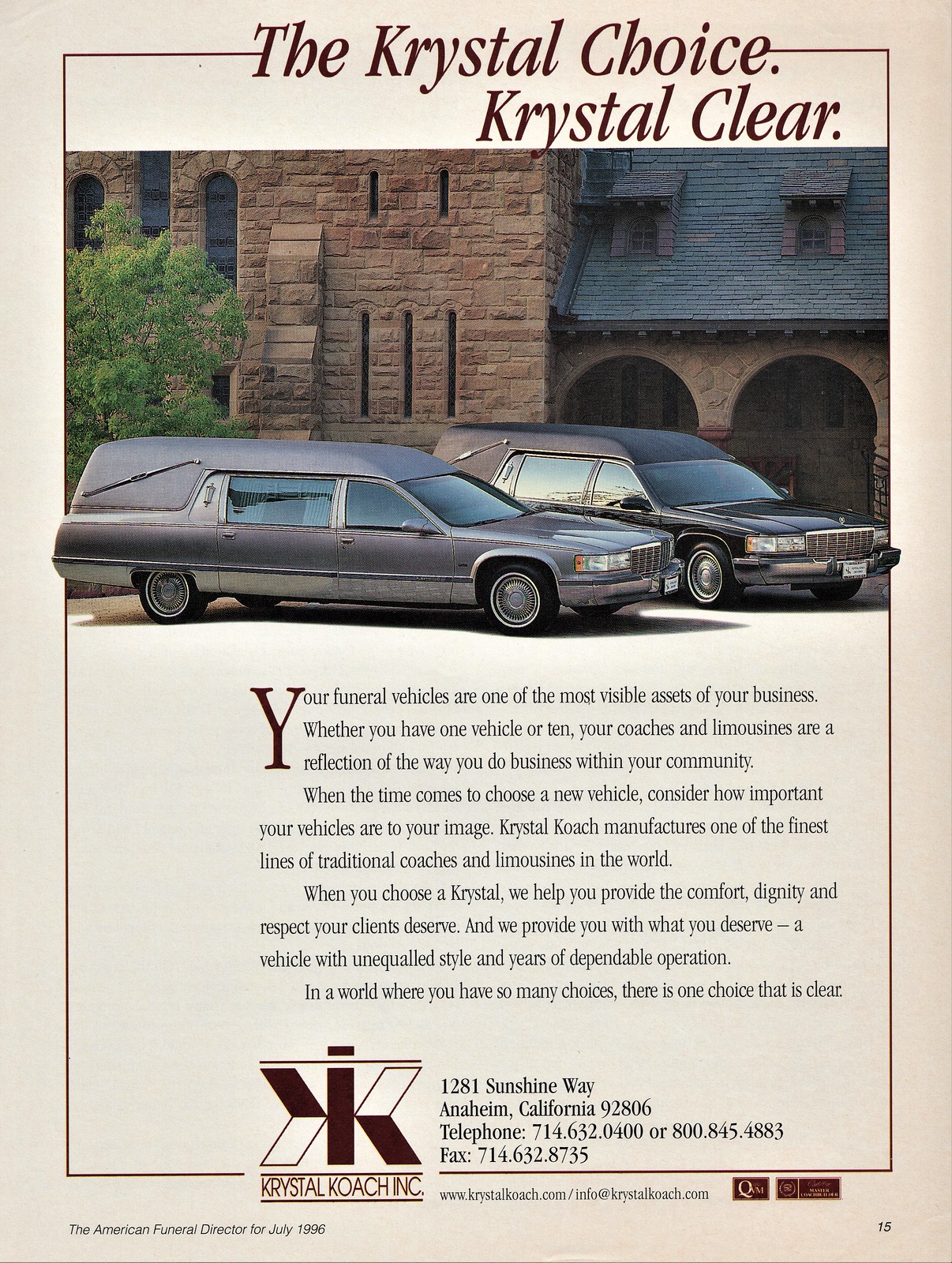This is a magazine advertisement for Crystal Coach Inc., showcasing two sleek gray and black hearses positioned in front of a substantial beige stone building. The building appears large and heavy, adding to the solemnity of the image. In the background, a gray-roofed stone church and a tree complete the scene.

At the top of the advertisement, bold text reads, "The Crystal Choice, Crystal Clear." Below the image, the ad emphasizes the importance of funeral vehicles as visible assets for funeral businesses, stating, "Your funeral vehicles are one of the most visible assets of your business. Whether you have one vehicle or ten, your coaches and limousines are a reflection of the way you do business within your community. When the time comes to choose a new vehicle, consider how important your vehicles are to your image."

Further down, it elaborates on the quality and reputation of the vehicles, "Crystal Coach manufactures one of the finest lines of traditional coaches and limousines in the world. When you choose a Crystal, we help you provide the comfort, dignity, and respect your clients deserve, and we provide you with what you deserve, a vehicle with unequaled style and years of dependable operation. In a world where you have so many choices, there is one choice that is clear."

At the bottom, the company’s logo—resembling two back-to-back Ks with a vertical bar in between, and the words "Crystal Coach INC"—is displayed alongside contact information.